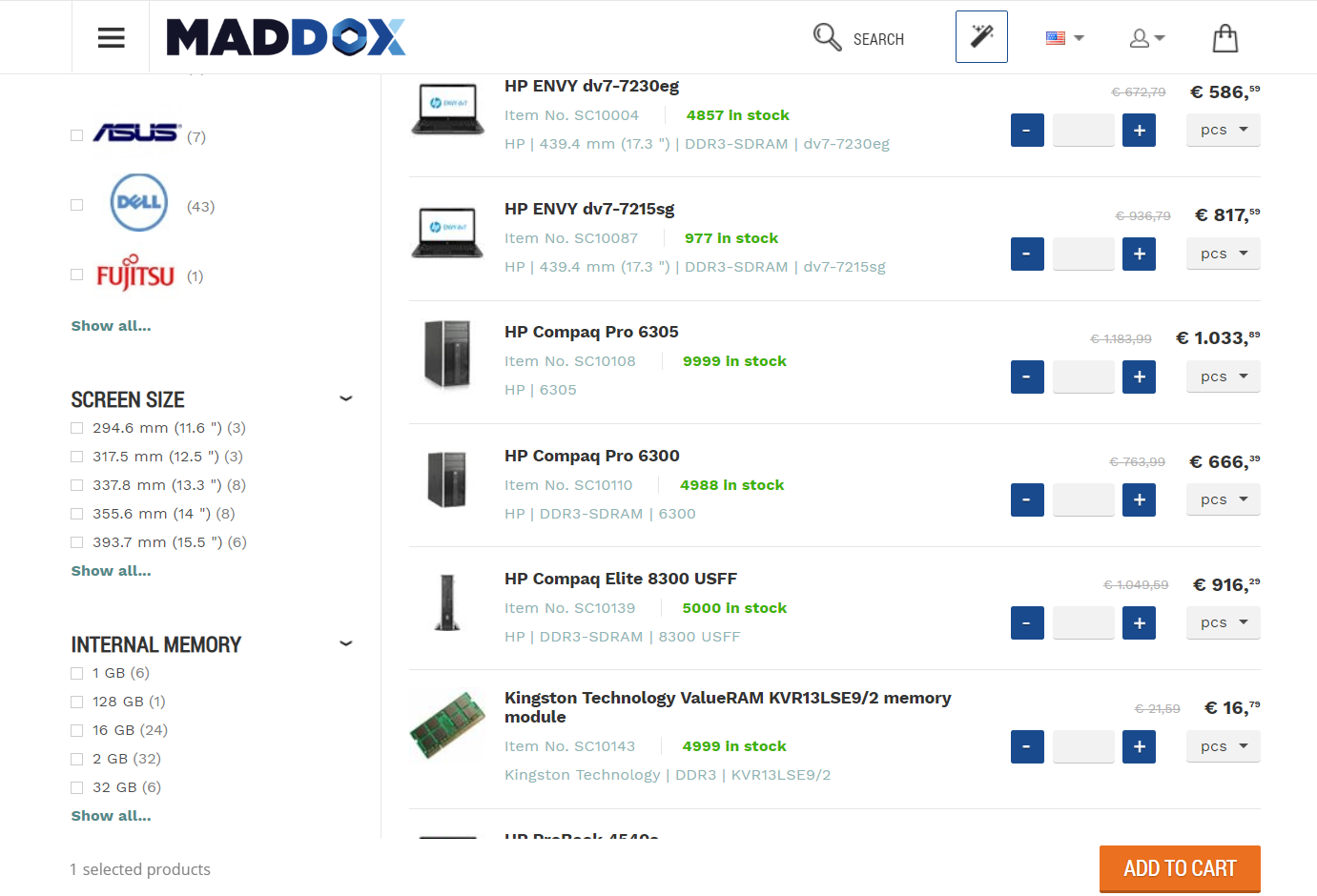The image depicts a detailed interface of an online shopping website for electronic brands and products. 

In the upper left-hand side, there is a white section featuring three black lines. Following this is the branding with the word "MAD" in black, and "DOCKS" in blue. Adjacent to this branding, a gray magnifying glass icon appears with the word "Search" grayed out next to it. Below this, there is a black and white wand icon, outlined in blue. Additionally, an American flag is present, depicted with a gray triangle pointed downward. Nearby, a gray triangle pointing downward and a gray shopping bag icon are displayed.

On the left-hand side, a list of different electronics brands is visible. The first brand listed is "Asus" in blue, followed by "Dell" also in blue. "Fujitsu" appears in red, and "Shuo..." in green. Below this, the text "Screen Size" is shown in black, listing the following measurements: 29.6 mm (11.6 inches), 317.5 mm, 337.8 mm, 355.6 mm, and 393.7 mm. The brand "Shuo" is repeated and highlighted in green, followed by the text "Eternal Memory" in black, with various capacities listed: 1 GB, 128 GB, 16 GB, 2 GB, and 32 GB. "Shuo..." is repeated once more in green, with the text "One Selected Products" in gray underneath.

To the right, another set of products is listed, starting with "HP ENVY." This is followed by "HP ENVY HP Compact Pro," "HP Compact Pro 6300," and "HP Compact Pro 6305." Next, "HP Compact Elite 8300USSFF" is listed. The last product mentioned is "Kingston Technology Value RAM."